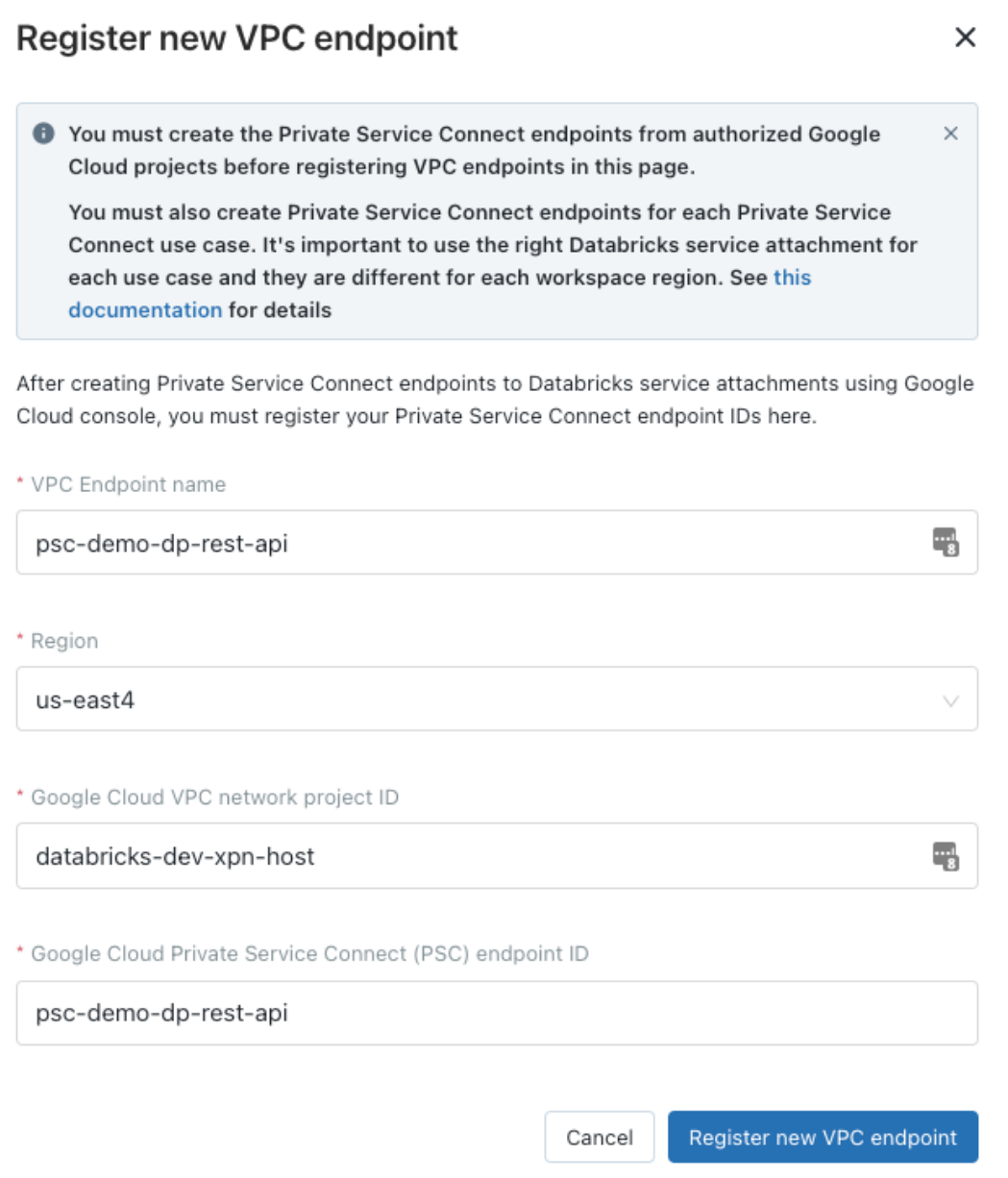This image depicts a registration page for creating a new VPC (Virtual Private Cloud) endpoint. At the top of the page, a prominent information box emphasizes the necessity of creating Private Service Connect endpoints from authorized Google Cloud projects prior to registering VPC endpoints on this page. The notice further details that separate Private Service Connect endpoints must be created for each specific use case, highlighting the importance of selecting the appropriate Databricks service attachments for each workspace region. A link to additional documentation, highlighted in blue, is provided for further details.

The lower section of the page includes fields where users can enter their private service endpoint IDs, a task that must be completed after generating Private Service Connect endpoints via the Google Cloud Console. The page is organized with various headings guiding users through the required information.

Once all fields are filled, users can proceed by clicking the blue "Register New VPC Endpoint" button at the bottom, finalizing the registration process.